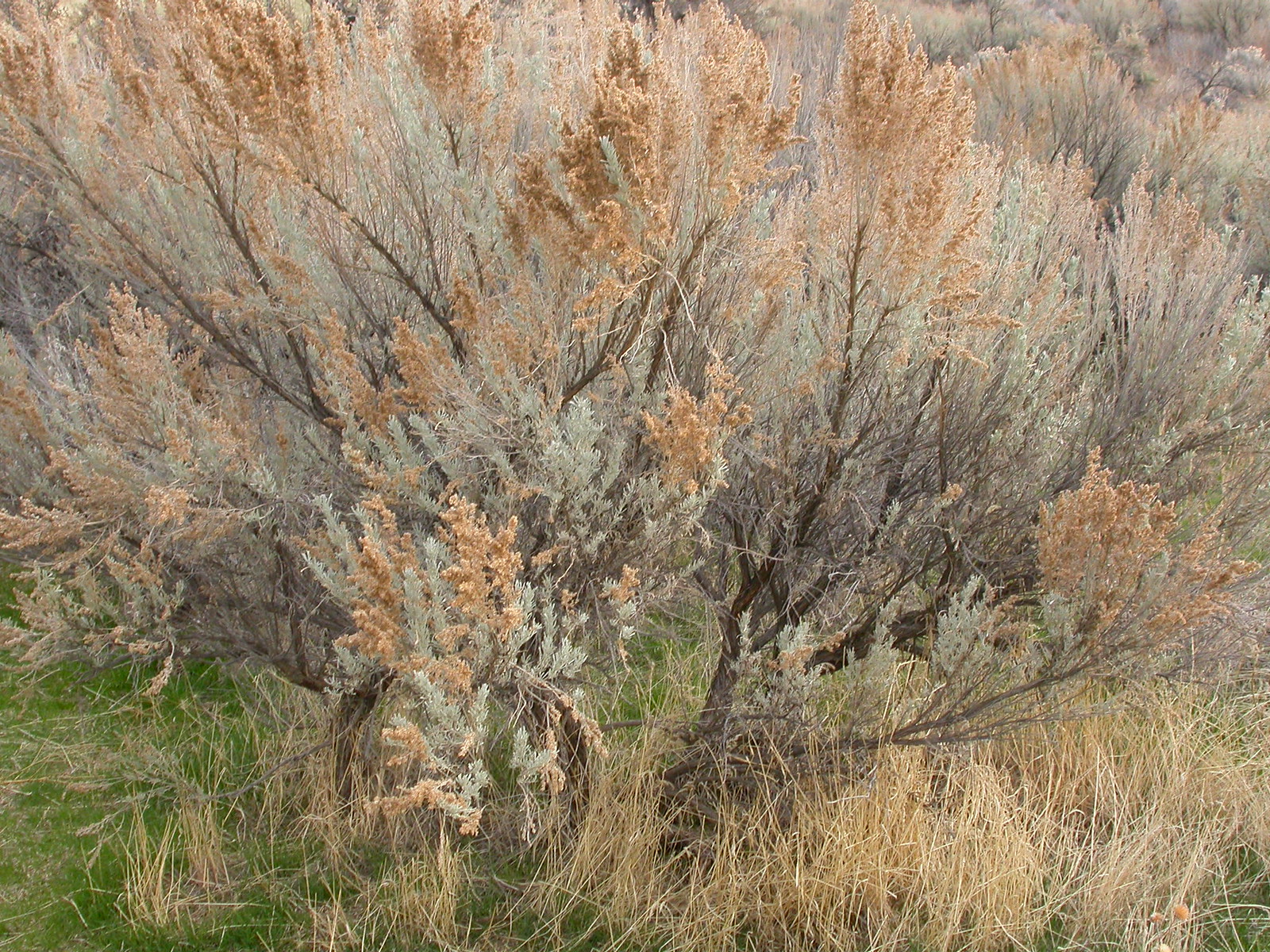In this outdoor photograph taken during the day, a small bush-like tree with a thin trunk stands prominently in the foreground. Multiple branches extend from the trunk, covered in both small white and brown leaves, creating a rustic, monochromatic look. The tree is surrounded by various strands of grass: tall yellowish-brown blades and much shorter green ones, interspersed with patches of bare dirt. The scene appears to be bathed in natural daylight, lending a slightly overcast or cloudy ambiance that highlights the dryness of the vegetation, suggesting a time in either late spring, summer, or early autumn. In the distance, similar small bushes or trees, also adorned with white and brown leaves, stretch across a slight slope, forming a dense, bushy area that recedes into the landscape. The overall impression is one of a dry, warm climate with a blend of vibrant, yet earthy tones and textures.